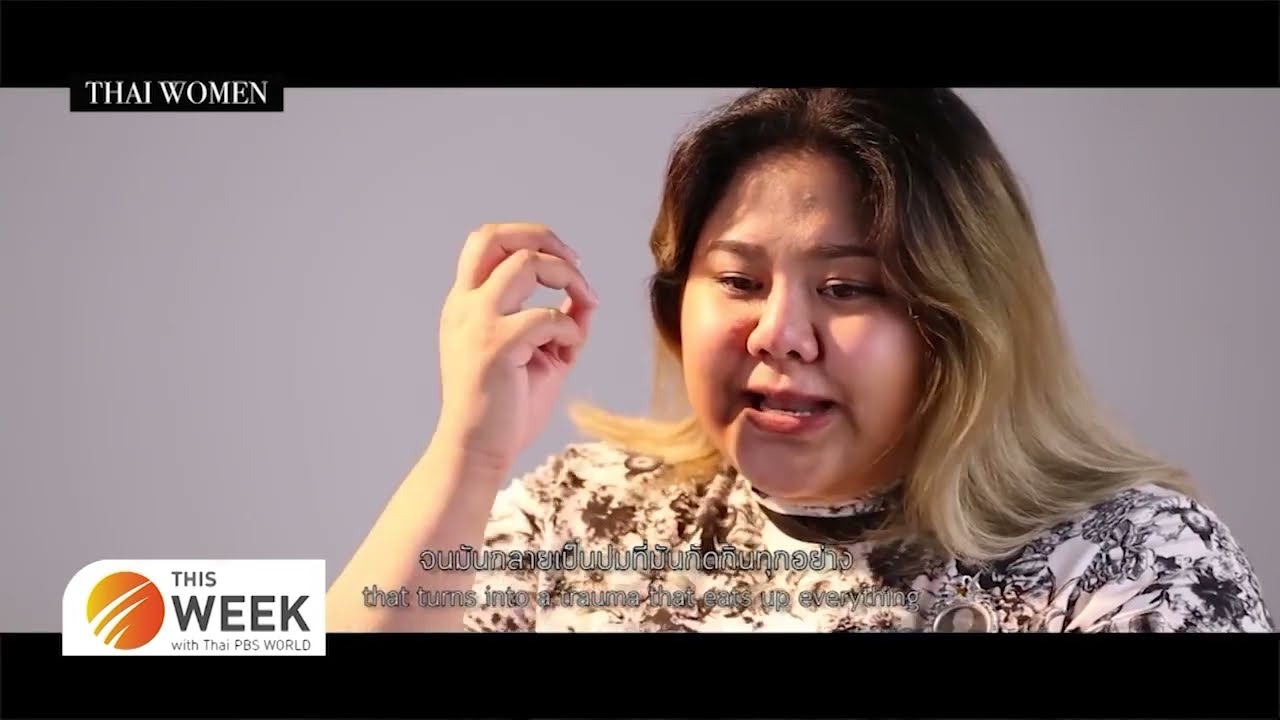The image is a still shot from a video, likely a news report or interview. It features a slightly overweight Thai woman with a round face and dark hair dyed blonde at the ends, showing some darker roots. She appears to be in mid-speech, gesturing with her right hand up to emphasize a point. The woman, wearing a black and white shirt with a floral pattern, is captured from the chest and shoulders up, looking downwards. The video has a thin black header and footer. In the upper left corner, white text on a black background reads "Thai Women." The lower right corner displays a logo in a white rectangle with a beveled edge, featuring an orange globe and the text "This Week with Thai PBS World." Below the woman, closed captioning is visible in Thai, with an English translation that reads, "that turns into a trauma that eats up everything." The screenshot is paused or screen-grabbed, giving the impression of a live moment frozen in time.